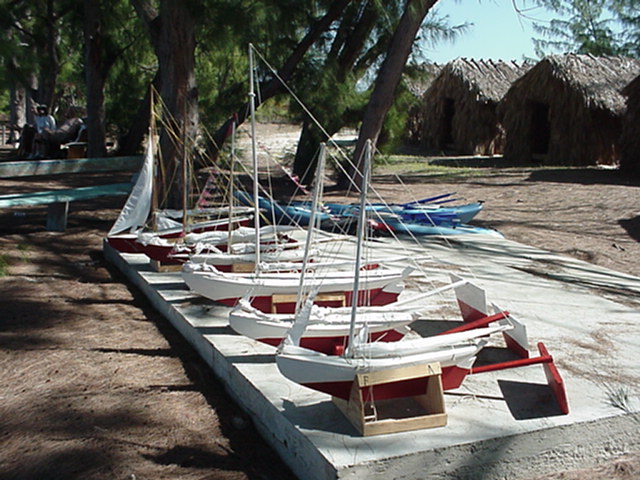In this photograph, six miniature scale sailboats designed for RC competitions are neatly lined up on a white concrete pad that is raised about eight inches above the dirt ground. Each boat is meticulously painted with a white top and red bottom, while one features a blue color. The sailboats, resembling typical sloops, are equipped with oversized rudders, and only one has its white sail unfurled. The boats are secured upright by large wooden supports on each side. The background reveals a series of brown thatch-roof huts and scattered trees, creating a shaded area beneath a clear blue sky. Additionally, what appears to be an on-ramp into a large pool is visible on the upper left side of the image, though slightly obscured. The vibrant scene captures a blend of natural and man-made elements, emphasizing the quaint yet detailed setup of the miniature regatta.